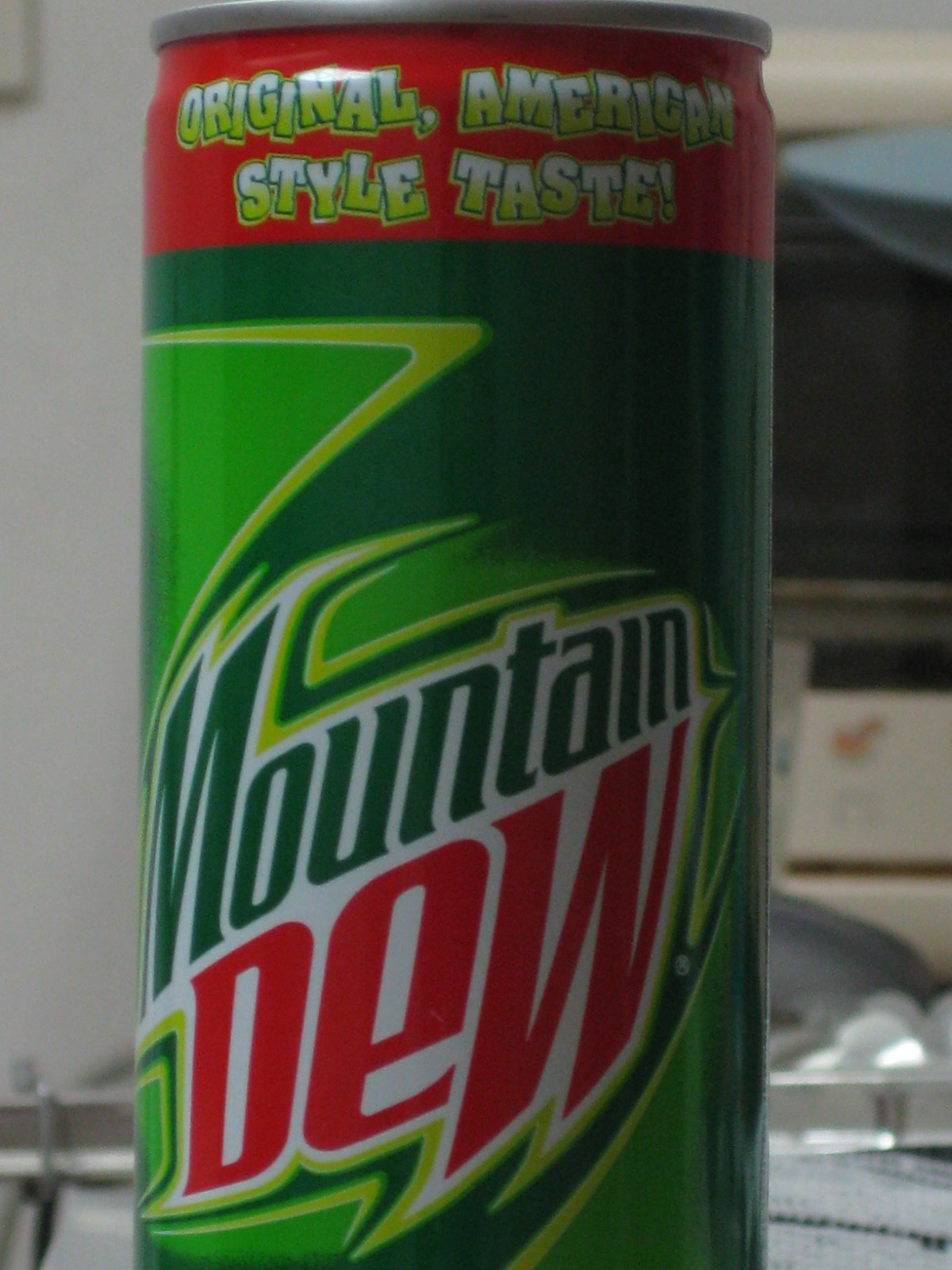A close-up shot captures a Mountain Dew can, focusing on the vibrant logo which features prominently in the center. The image is tightly cropped, cutting off the very top where the tab would be and the bottom edge of the can. The "Mountain Dew" logo, in its signature bold red and green font, is the central element of the composition. Above the logo, the phrases "Original" and "American Style Taste" are visible in a green font with a white outline. The can appears to be placed on a countertop, with a white towel partially visible in the bottom right corner behind it. The overall setting suggests a casual, everyday environment, enhancing the familiar appeal of the Mountain Dew brand.